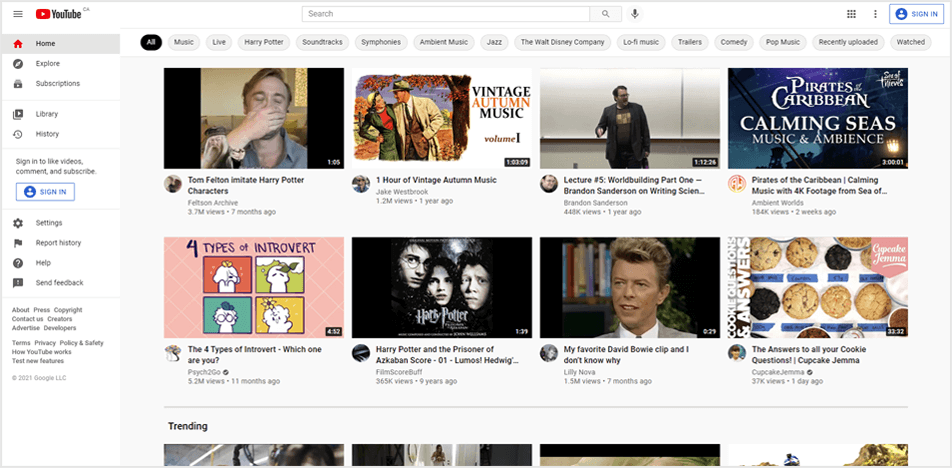Screenshot of YouTube Homepage with Detailed Menu and Video Thumbnails

In this YouTube screenshot, the iconic YouTube logo featuring a red rectangle with a white play button sits prominently in the top left-hand corner. Adjacent to this, a horizontal search bar awaits user input, flanked by a microphone icon, a three-dot menu, and a tiny blue account picture labeled "Sign in," all situated on the top right-hand side. 

Moving to the left-hand side, the interface displays a vertical menu beginning with a red-highlighted "Home" button. Beneath this are options such as "Explore," "Subscriptions," "Library," and "History." Further down, users can see "Sign In," "Settings," "Report History," "Help," and "Send Feedback."

Across the top of the main interface, a secondary horizontal menu categorizes videos into sections like "All," "Music," "Live," "Harry Potter," "Soundtracks," "Symphonies," "Ambient Music," "Jazz," "Walt Disney Company," "Lo-fi Music," "Trailers," "Comedy," "Pop Music," "Recently Uploaded," and "Watched."

Below this, eight video thumbnails capture immediate attention, each accompanied by descriptive titles:
1. "Tom Felton Imitates Harry Potter Characters" with an image of an actor.
2. "One Hour Vintage Autumn Music."
3. "Lecture Number Five: Word Building."
4. "Pirates of the Caribbean Calming Sea Music."
5. "Four Types of Introverts."
6. "Harry Potter: Prisoner of Azkaban Score."
7. "My Favorite David Bowie Clip."
8. "Answer to All Your Cookie Questions" featuring a picture of an assortment of cookies.

This comprehensive interface provides a seamless navigation experience, appealing to a wide range of user preferences and interests.